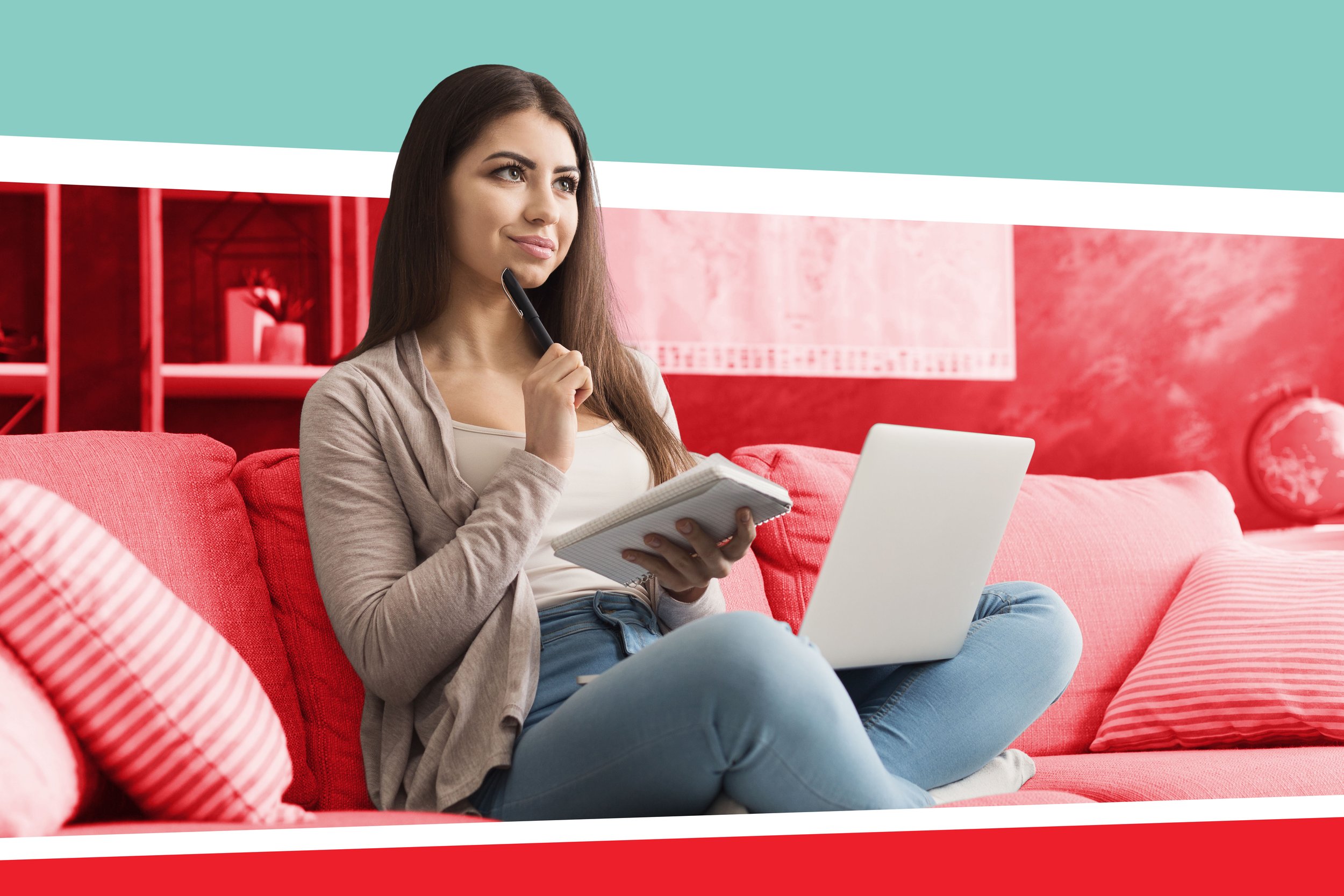In this photograph, a young woman, appearing to be in her mid-20s to 30s, with long, straight brown hair parted in the middle and striking green-blue eyes, is deeply engrossed in thought. She is seated cross-legged on a bright pink couch adorned with striped white and pink cushions. Dressed comfortably in a white crop top, a tan pullover sweater, and light blue jeans, she holds a white notepad in her left hand and a black pen in her right hand, with the pen's tip touching the right side of her chin. Her white laptop rests on her lap. Behind her, the wall features a split design: the upper half is a light turquoise, while the lower half matches the bright pink of the couch. This setting, coupled with the thoughtful pose of the woman, gives the impression that she is deeply contemplating or brainstorming, potentially for an advertisement or promotional image.